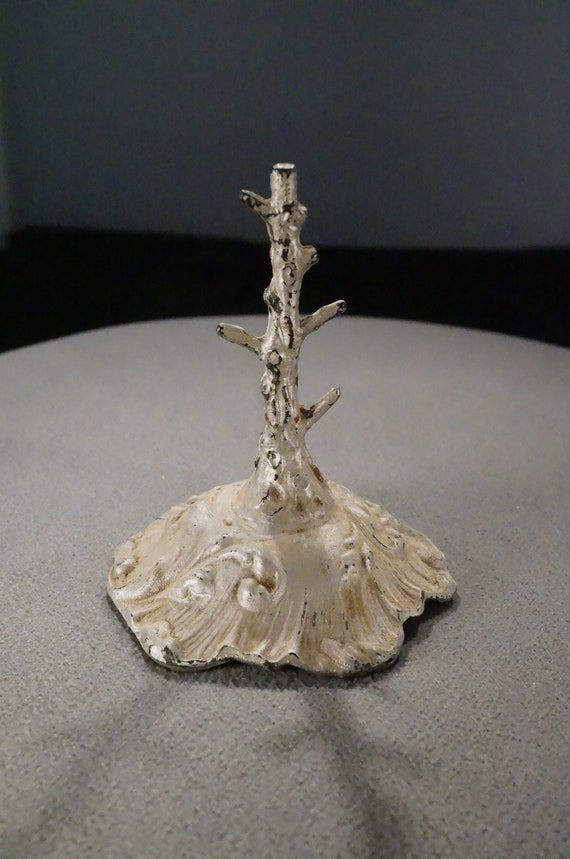The image depicts an artistic sculpture that intricately combines elements of both wood and ceramic design. The centerpiece is a textured, pearl-colored base reminiscent of an upside-down flower, beautifully reflecting white and yellowish hues. This base, detailed with numerous lines and curves, elevates into a tree trunk-like structure adorned with small nubs mimicking branches. The sculpture appears aged and slightly tarnished, featuring blackened areas that suggest it was once completely white. It rests on a light gray surface, possibly a circular rug or a table, while the background is stark black, accentuated by a light source creating a reflective shadow that extends down to the left. The piece, evoking the image of a barren, leafless tree, presents a unique and interesting blend of textures and forms, making it both a visual and tactile work of art.